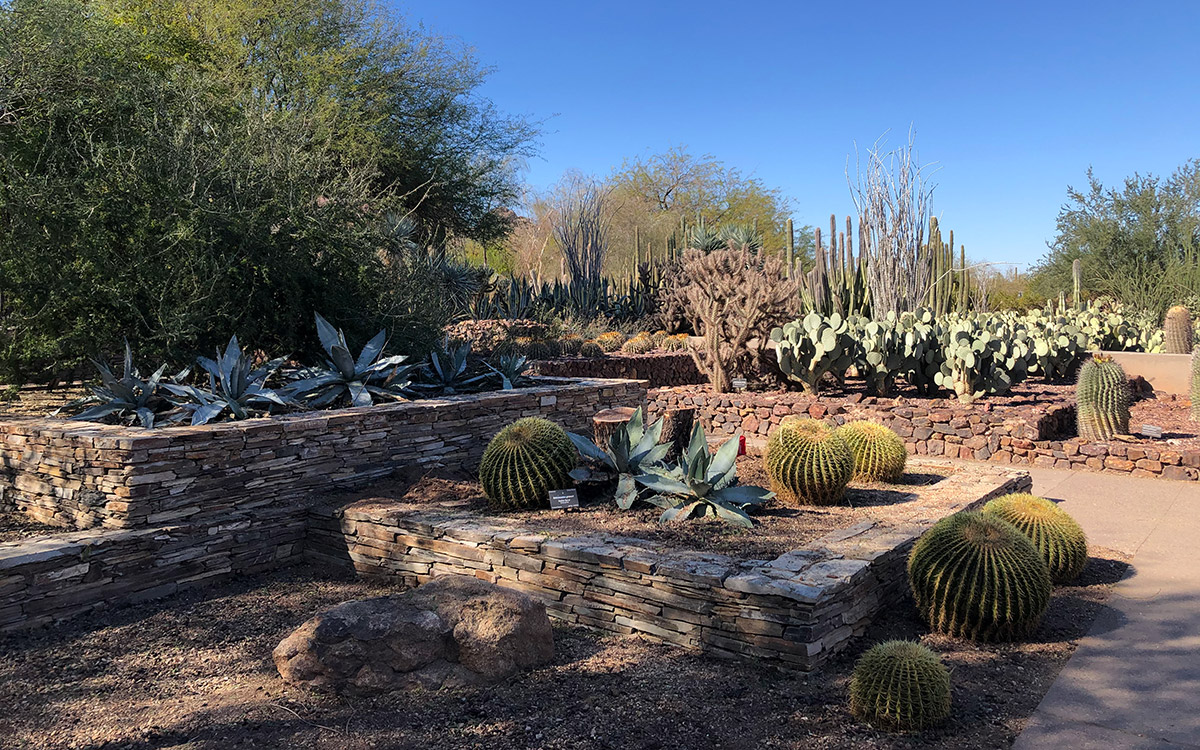The image appears to depict a desert-themed park, abundant with various types of cacti. At the center of the picture, there is a raised square brick platform, meticulously landscaped, surrounded by round cacti. To the left, the terrain elevates further, hosting additional cacti and a prominent bush or small tree. Straight ahead, the brick landscaping continues, leading the eye to a seemingly endless expanse filled with an impressive assortment of cacti stretching out to the horizon.